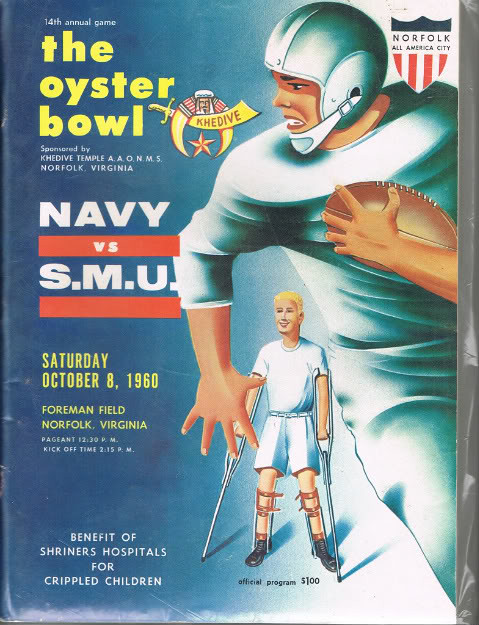The image is the front cover of an official sports magazine or program from the 14th Annual Game, the Oyster Bowl, held on Saturday, October 8, 1960, at Foreman Field in Norfolk, Virginia. The event, sponsored by Khedive Temple, A-A-O-N-M-S, and benefiting Shriners Hospitals for Crippled Children, features a football match between the Navy and SMU. The cover is dominated by a detailed and colorful illustration of a football player in a green jersey and helmet, carrying a football against his chest. Behind this player is a small child with blonde hair wearing a white t-shirt and shorts, using crutches and leg braces similar to those worn by Forrest Gump as a child. The cover prominently displays text in blue, yellow, white, red, gray, light blue, and green, indicating the event details, including the kickoff time at 2:15 p.m. and the price of the program at $1.